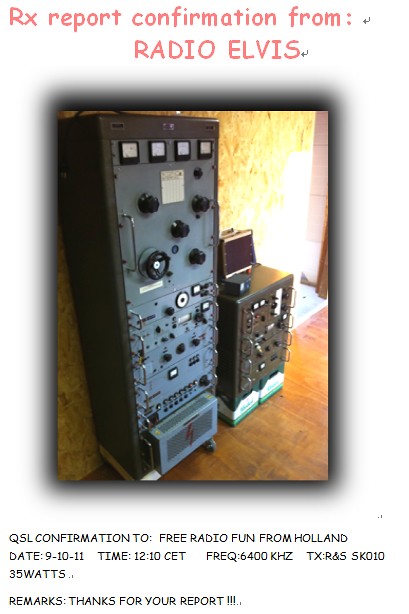The thank you card features a stark white background with prominent red text at the top that reads "RX Report Confirmation from Radio Elvis." Below this text, there is a photograph resembling an old Polaroid, displaying a large, tall, gray radio transmitter that looks like antique machinery. This device is fitted with various analog sensors, knobs, buttons, and gears, resembling a tall cabinet, accompanied by a shorter cabinet with a screen on the top, suggesting a detailed electronic setup. The floor beneath the equipment is brown, and the wall behind it is yellow. Below the photograph, there is black text stating, "QSL Confirmation to Free Radio Fund from Holland. Date 9-10-11, Time 12:10 CET, Frequency 6400 kHz, TX RNS SK 010, 35 watts. Remarks: Thanks for your report."